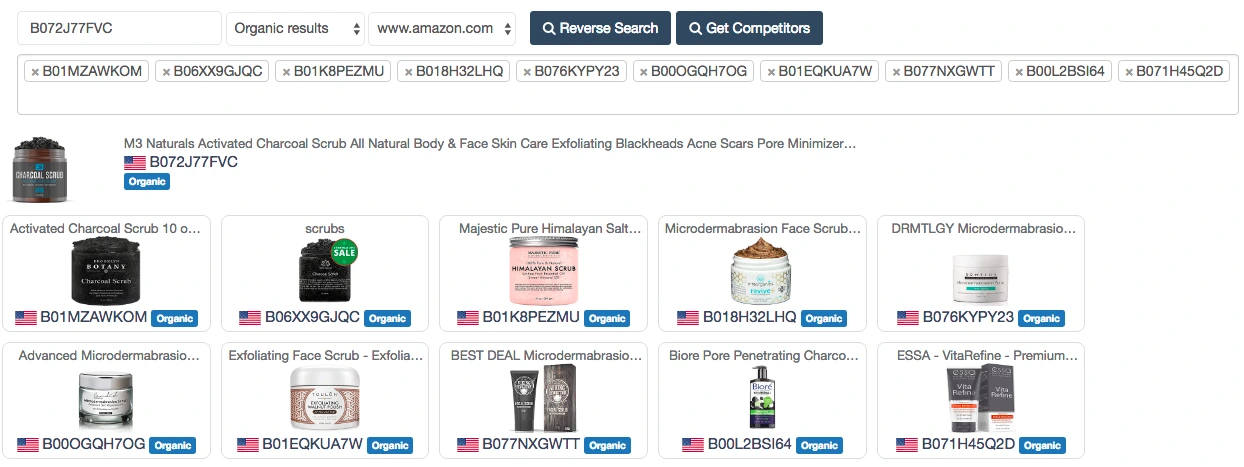Screenshot of search results displayed under a platform labeled "Flavors Search" with an option "Get Competitors" in blue. The search reference number given is B072J77FVC. Below that, organic search results from www.amazon.com are listed showcasing images and descriptions of several skincare products:

1. **M3 Natural Activated Charcoal Scrub** - Presented in a black container, this product promises all-natural body and face skincare benefits, including exfoliation to target blackheads, acne, and pores, while minimizing their appearance.
2. **Activated Charcoal Scrub 10** - Enclosed in a similar black container, this scrub carries organic certification from the USA.
3. **Majestic Pure Himalayan Salt Scrub** - Also labeled as organic and produced in the USA, this scrub offers microdermabrasion benefits for the face.
4. **Dermatology Microdermabrasion Face Scrub** - Marketed as an organic product from the USA, meant for facial exfoliation.
5. **Advanced Modern Organic** - Another entry in the organic skincare category.
6. **Exfoliating Face Scrub** - Final product in the listing, also highlighted for its organic features.

All items are highlighted as organic, predominantly from the USA, emphasizing various exfoliating and skincare benefits.